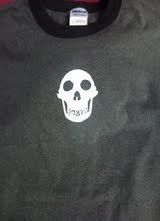A crisp, dark gray t-shirt is neatly laid out, showcasing a striking design at the center. The neck lining is a solid black, accentuating the garment's sleek appearance. A white label is embedded in the collar, though its text remains unreadable. The focal point of the t-shirt is a small, intricately designed skull. The skull features rounded eye sockets and a uniquely shaped nose, with teeth that resemble more of an ape than a human. This distinctive graphic stands out against the smooth, flat fabric of the shirt, creating a minimalist yet captivating visual appeal. No additional text or logos are present, emphasizing the bold simplicity of the design.